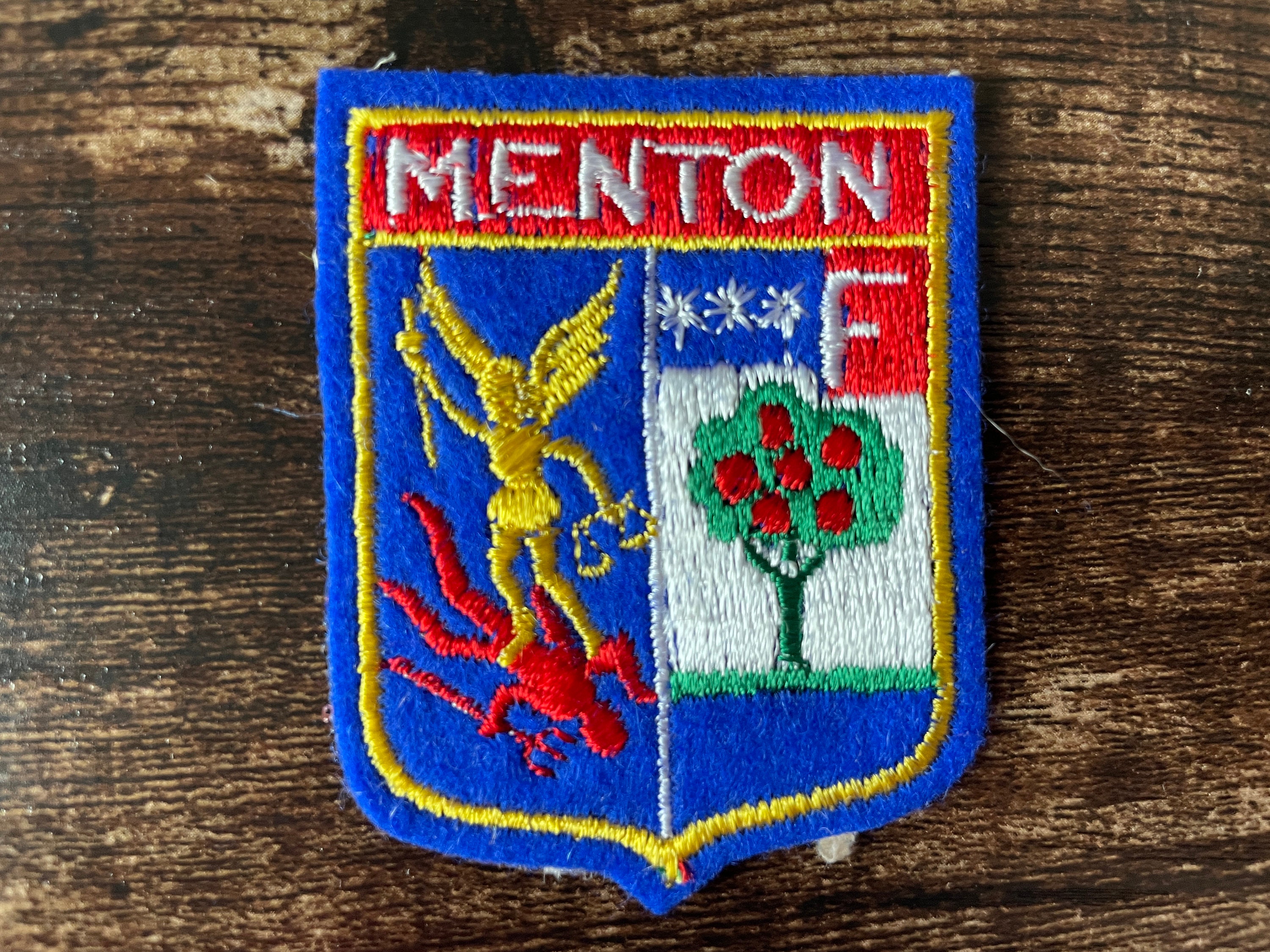The image showcases an up-close shot of a vibrant blue patch shaped like a shield, resting on a rustic wooden surface. The patch is richly bordered with a golden outline and features a red top bar displaying the word "Menton" in white stitching. On the left side of the patch, a golden angel is depicted triumphantly standing over a red devil carrying a pitchfork. The angel, in a dynamic pose, holds a sword raised as if ready to swing and a pair of scales representing justice in the other hand. The right side of the patch displays an apple tree with red fruits against a white background, accompanied by the letter "F" in a red rectangle. Above the tree, three white stars are set against a blue backdrop, completing the intricate design of the patch.